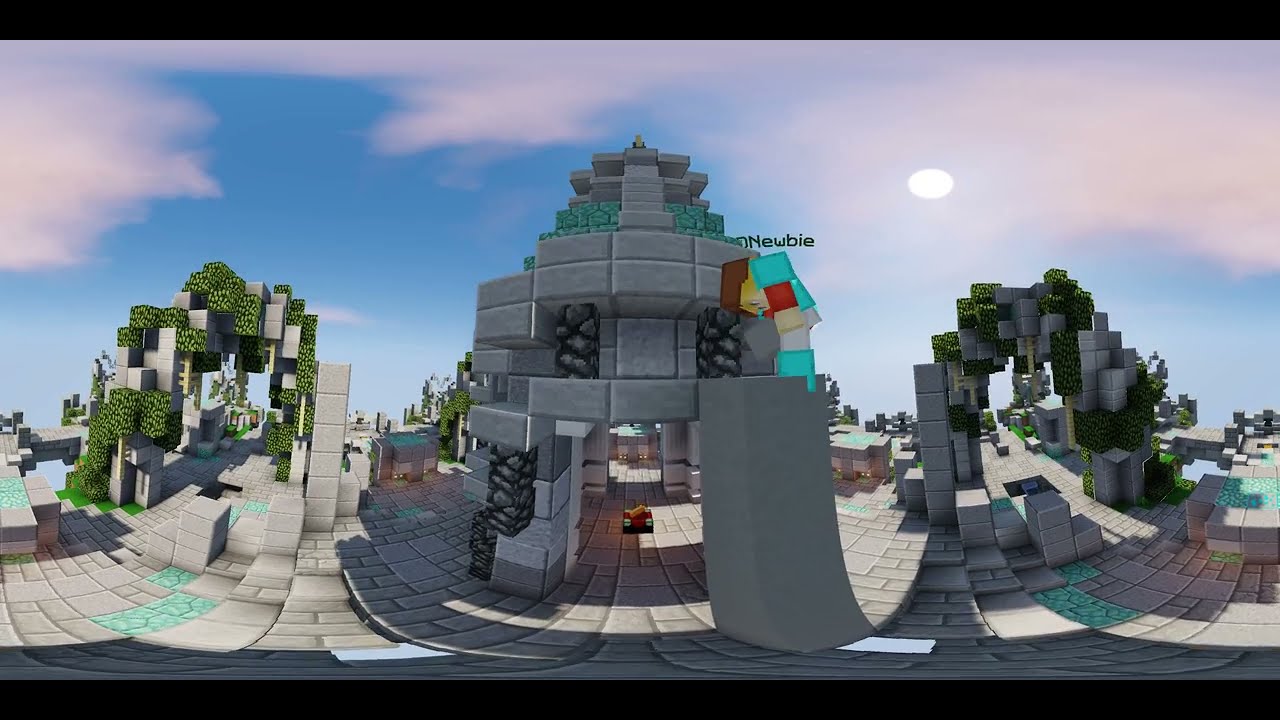The image depicts a vibrant Minecraft scene with three floating islands set against a bright blue sky dotted with pinkish-white clouds and a radiant yellow sun on the left. The central island, the largest and nearest to the viewer, is composed mainly of grass, stone, and cobblestone blocks. It features two facing chests and a statue shaped like a heart on its surface. Hovering above this statue is a multicolored cross constructed from yellow, red, and green blocks. To the right of the central island, there's another floating structure adorned with cobblestone, grass, and dirt, and a distinctive ladder or cage-like formation suspended above it. The leftmost island, mainly a mass of cobblestone, also includes dirt blocks and a tree. All three islands convey the quintessential Minecraft aesthetic, complete with blocky textures and a digitally-rendered charm. The scene evokes a sense of whimsy and adventure, characteristic of the game.